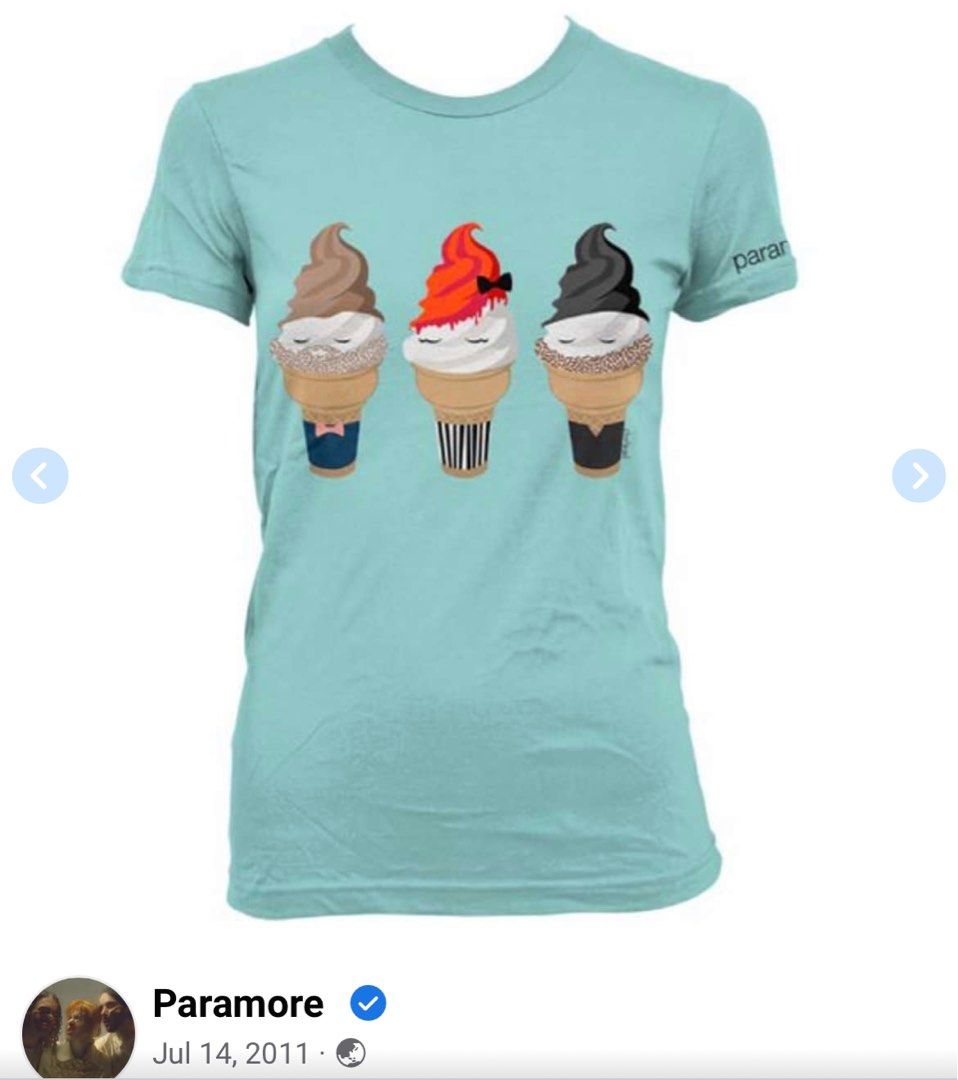This image displays a turquoise crew neck t-shirt with short sleeves, adorned with three quirky ice cream cone characters on the front. Each ice cream cone features eyes and a unique swirled topping that resembles hair, possibly stylized to match members of the band Paramore. The leftmost cone has a brown swirl resembling hair and a beard, with blue wrapping around its base and a pink area mimicking a bowtie. The middle cone has a red swirled hair with a black bow, and is wrapped in black and white vertical stripes. The rightmost cone sports a black hair swirl and brown beard, with a black wrapping resembling a vest. At the bottom of the shirt, the text "Paramore" is displayed in black, alongside a blue circle with a white check mark. Below this, the date "July 14, 2011" is printed. Additionally, there is a small, dark profile picture circle to the left, which seems to show an image of three people but lacks clear detail. The sleeve on the right side of the shirt also features black text that reads "P-A-R-A" but is partially cut off due to its curvature around the arm.